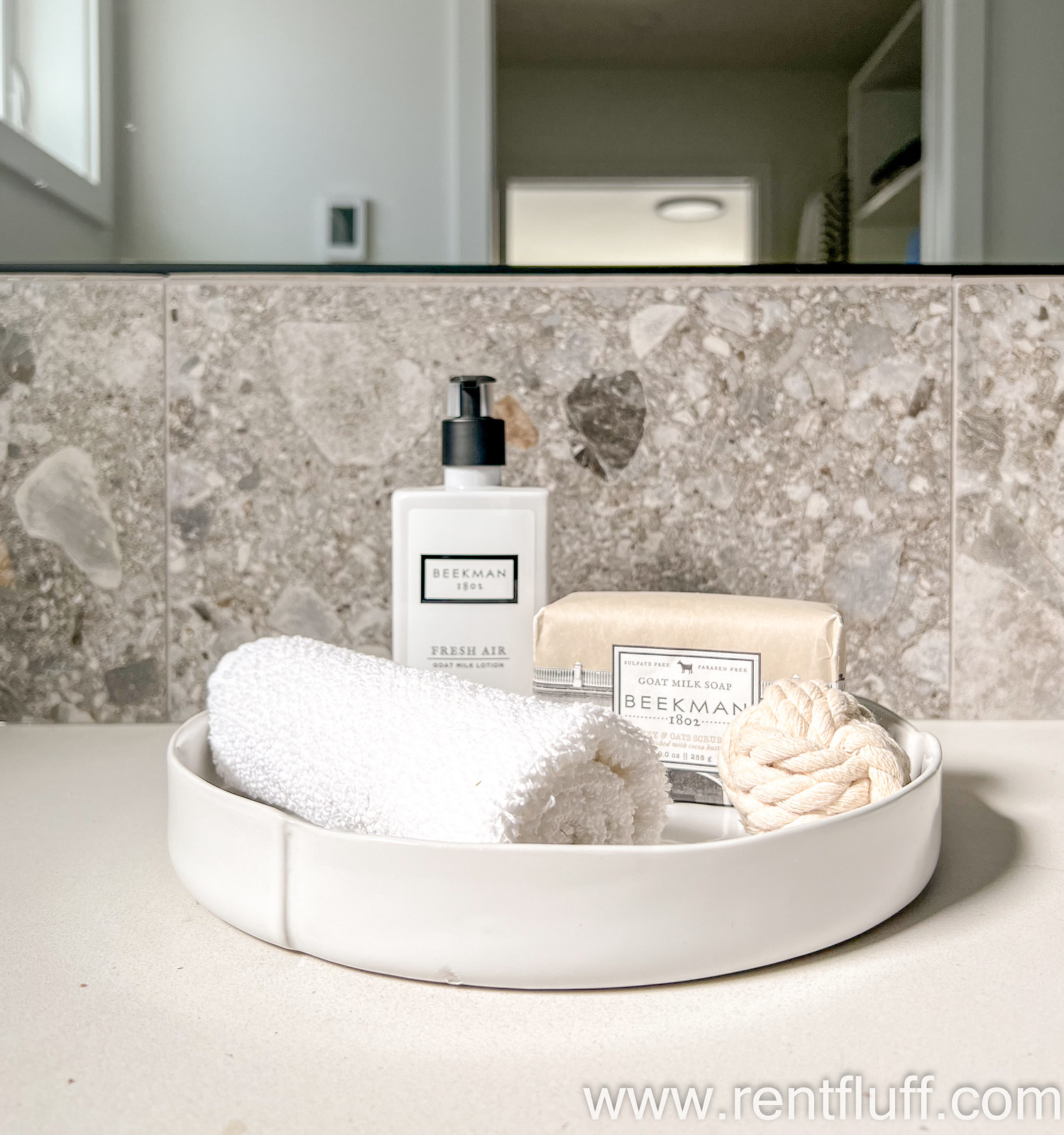This photograph showcases a meticulously arranged bathroom counter. Positioned at the bottom right corner, a pristine white countertop anchors the scene. The countertop is minimally adorned, enhancing the clean aesthetic.

Behind the counter, glossy square tiles—resembling either marble or granite—adorn the wall, adding a touch of elegance to the setting. A large mirror above these tiles reflects additional elements of the bathroom: a white door, several windows, and shelves, all contributing to a bright and cohesive space.

On the countertop itself, a round white container with low sides is visible; its material is ambiguous, possibly fabric or plastic. Nestled within this container is a neatly rolled washcloth. To its right lies a substantial knotted rope, adding a rustic element.

A prominently featured product is a dispensed bottle of Beekman 1802 Fresh Air, whose label is partially obscured. Adjacent to the bottle is a bar of Beekman 1802 goat milk soap, wrapped in tissue-like waxed paper, with its branding and weight in ounces or grams subtly noted on the packaging.

In the corner of the photograph, text on the countertop reads www.rentfluff.com, suggesting a rental service or staged setup, completing this organized and aesthetically pleasing bathroom scene.